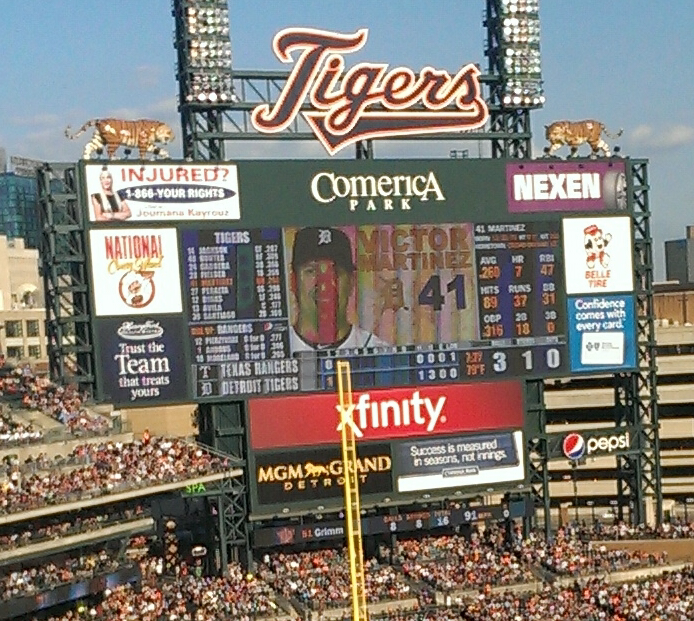This detailed photograph captures the bustling atmosphere of Comerica Park, home to the Detroit Tigers baseball team. The image prominently features the large, illuminated scoreboard and stands filled with spectators. Dominating the top of the scoreboard in a bold, blue, white, and red script is the word "Tigers," flanked by two metallic tiger statues, giving the impression of them prowling towards the emblem. Two towering floodlights stand on either side, ready to light the field for evening games. Below the Tigers logo, various advertisements are visible, including prominent ones for Xfinity and MGM Grand Detroit, alongside banners with sponsor names and motivational slogans like "Success is measured in seasons, not innings." The scoreboard also displays a picture of player Victor Martinez, denoted by his designation "D-41" and accompanied by his stats. The name "Comerica Park" crowns the scene in a sweeping banner, confirming the iconic venue.